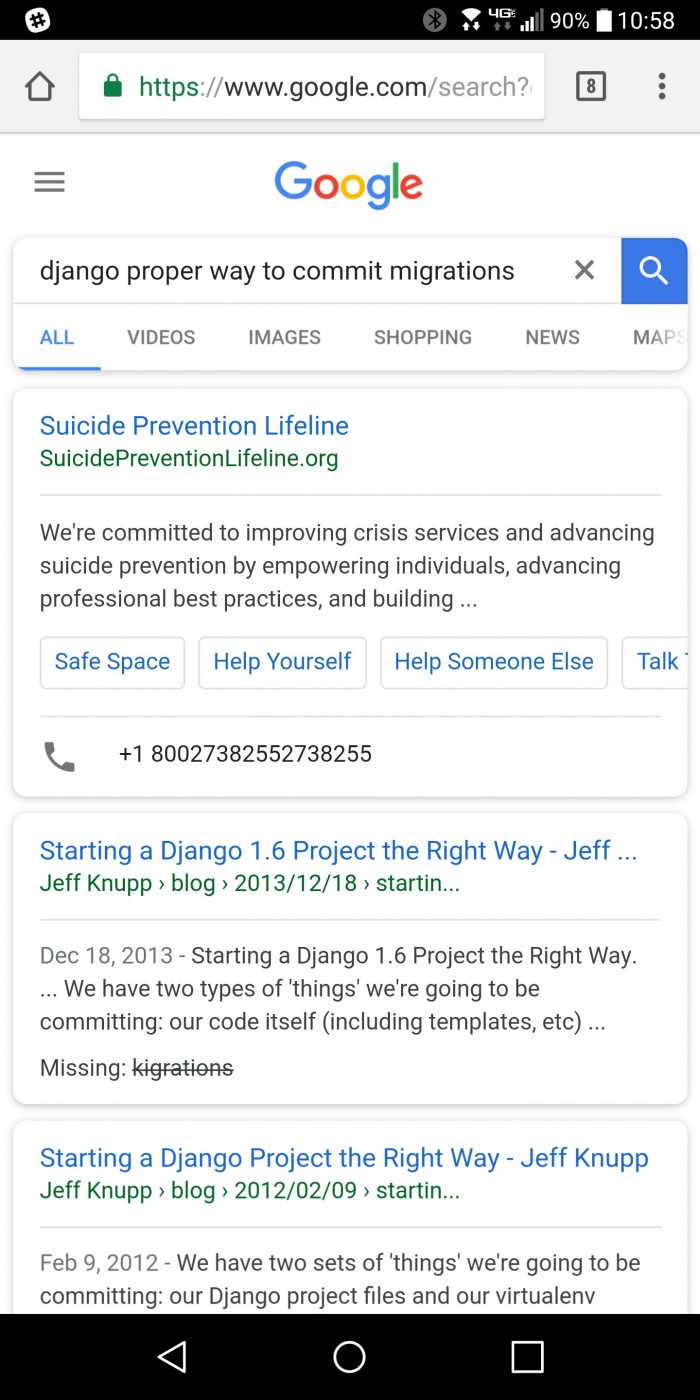The image depicts a Google search results page displayed on a smartphone. In the top left, there is a small white pound icon, and in the upper right, standard smartphone status indicators are visible, including a Bluetooth symbol, a 4G connectivity icon, a reception signal indicator, a Wi-Fi symbol, and a battery icon showing 90% with the time 10:58 displayed nearby. 

At the very top of the screen, the address bar features an '8' within a box, followed by the word "Google" in the familiar Google font. The search query "Django proper way to commit migrations" is entered in the search box beneath, accompanied by an 'X' button for clearing the input and a blue button with a white magnifying glass icon for initiating the search.

Immediately under the search box, several navigation tabs are presented, including "All," "Videos," "Images," "Shopping," "News," and "Maps." The first search result featured is for the "Suicide Prevention Lifeline," highlighted in blue with its URL "suicidepreventionlifeline.org" in green underneath, followed by a brief descriptive paragraph about the service. The subsequent search results include an entry titled "Starting a Django 1.6 Project the Right Way" and another one titled "Starting at the Django Project the Right Way" attributed to Jeff Nup.